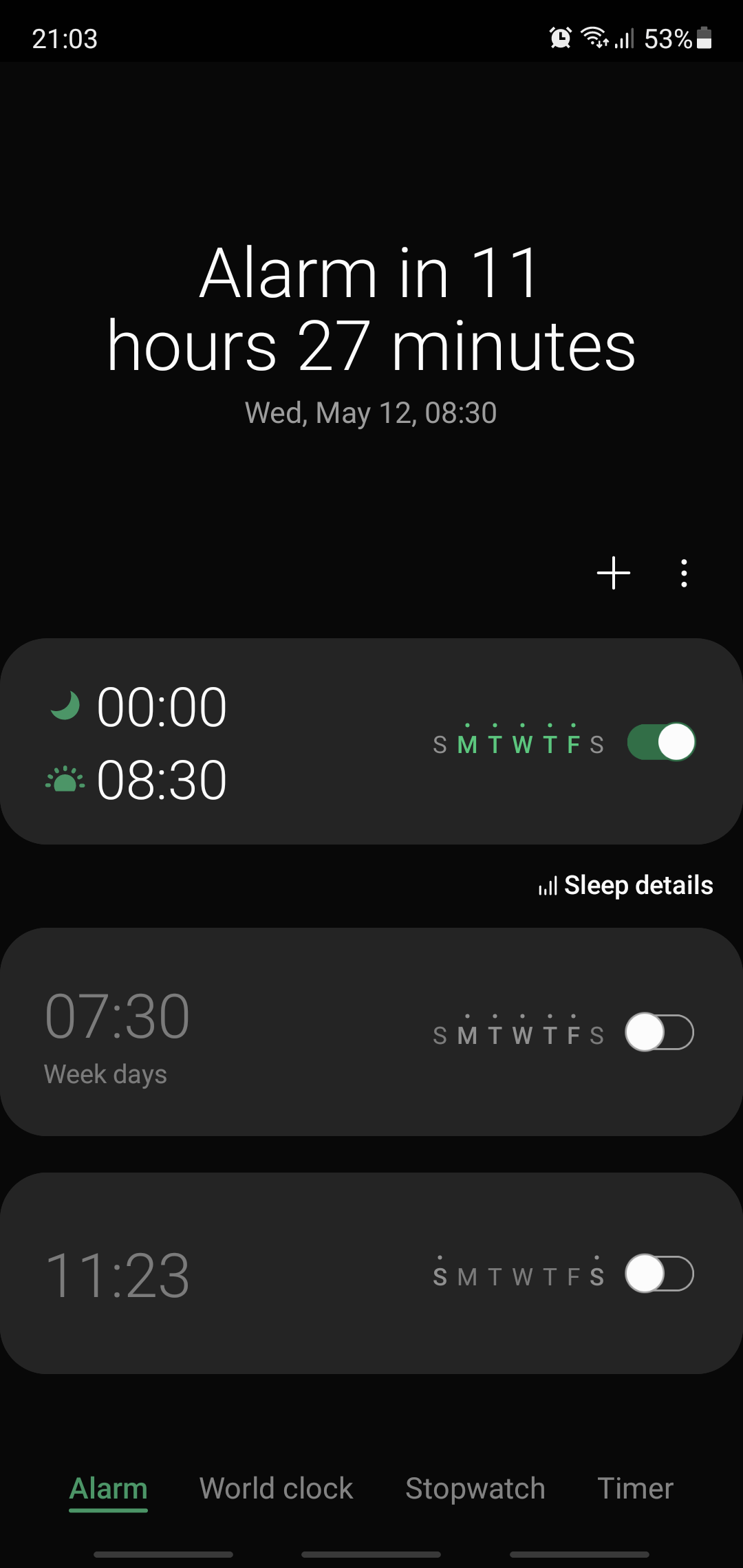This screenshot showcases the Alarms section of a smartphone against a black background with white font. The time displayed at the top left is 21:03. On the top right, the status bar shows full network connectivity with five bars, 53% battery life with a half-full battery icon.

At the center, there's a notification indicating the next alarm is set for 11 hours and 27 minutes from now, scheduled for 8:30 AM on Wednesday, May 12th. Below this, a plus sign and three dots provide options to add new alarms or access additional settings.

The first charcoal gray bar on the right side shows the "Bedtime" settings. A green moon icon marks the bedtime at midnight (00:00), and a green sun icon indicates the wake time at 8:30 AM. The selected days for this alarm, Monday through Friday, are highlighted in green, with the toggle switch in the 'on' position. Below this, an option labeled "Sleep Details" is present, allowing the user to view more information about their sleep patterns.

The second alarm setting in another charcoal gray bar displays an alarm set for 7:30 AM on weekdays. However, this alarm is currently turned off, as indicated by the inactive toggle switch and the non-highlighted initial letters of the days of the week.

The final charcoal gray bar lists another alarm set for 11:23 AM, with the days of the week shown but not selected or active, as the toggle bar is not turned on.

At the bottom of the screen, there are four navigation options: Alarm (which is currently in use and underlined in green), World Clock, Stopwatch, and Timer.